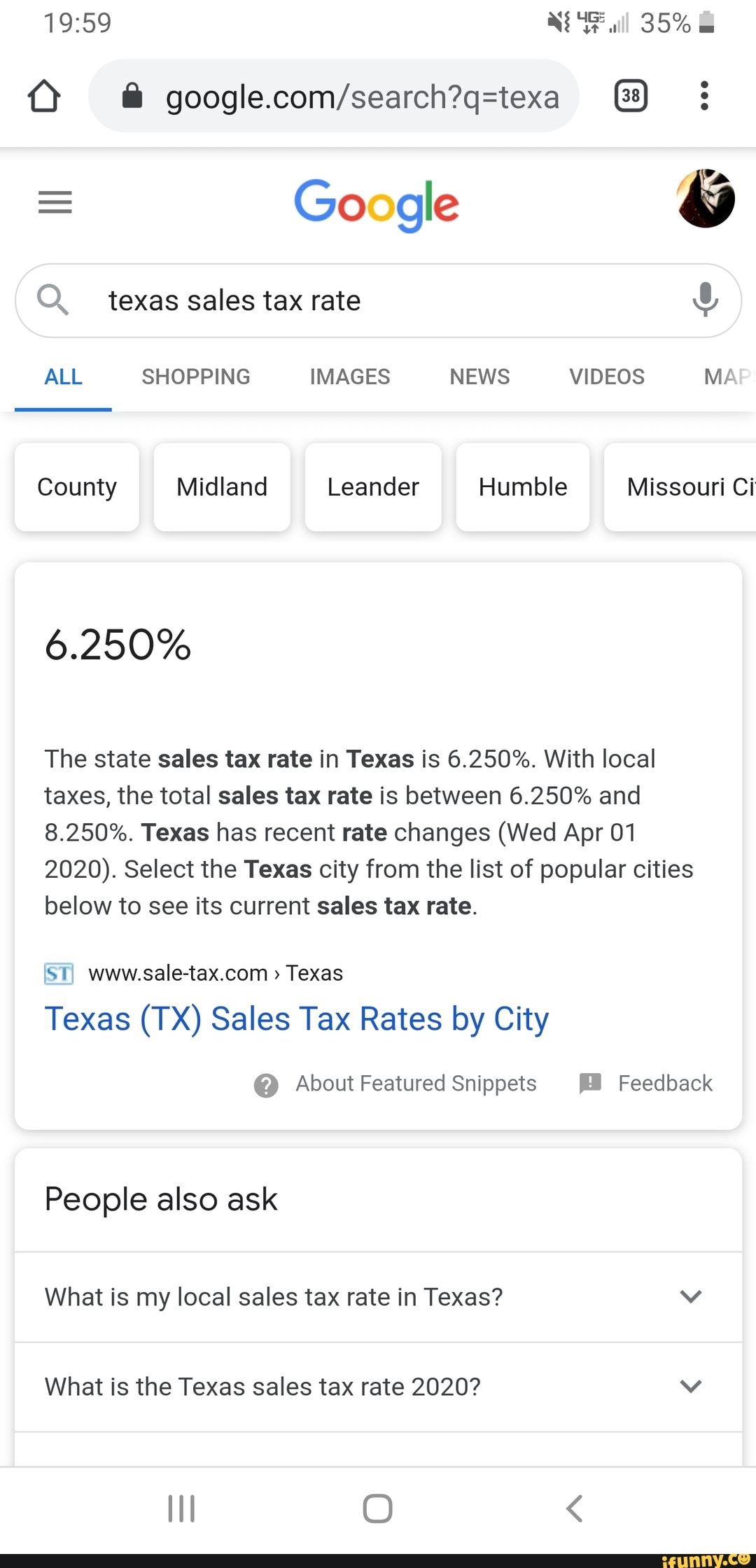This image is a screenshot of a phone displaying a Google search results page on a browser. At the top of the screenshot, the status bar shows the current time, a muted icon, a 4G connection, the cell signal bars, 35% battery life, and the battery icon. Below the status bar, the Google search interface is visible.

The search bar at the top contains the query "sales tax rate." Below the search bar, the Google logo is positioned at the top center of the main content area. To the left of the logo is a burger menu icon, and to the right, there is a profile picture.

Further down, the categories for filtering search results—'All,' 'Shopping,' 'Images,' 'News,' 'Videos,' and 'More'—are partially visible, extending off the screen to the right. Underneath these filters, boxed text appears, labeled left to right with "county," "Midland," "Lander," "Humboldt," and the partially visible word "Missouri."

A white box displaying "6.250%" follows, accompanied by explanatory text detailing the state sales tax rate in Texas. Below this text, a page link is provided. Another white box appears beneath it, labeled "People also ask," listing several related questions commonly asked by other users.

Lastly, the bottom of the screenshot includes the cell phone navigation icons.